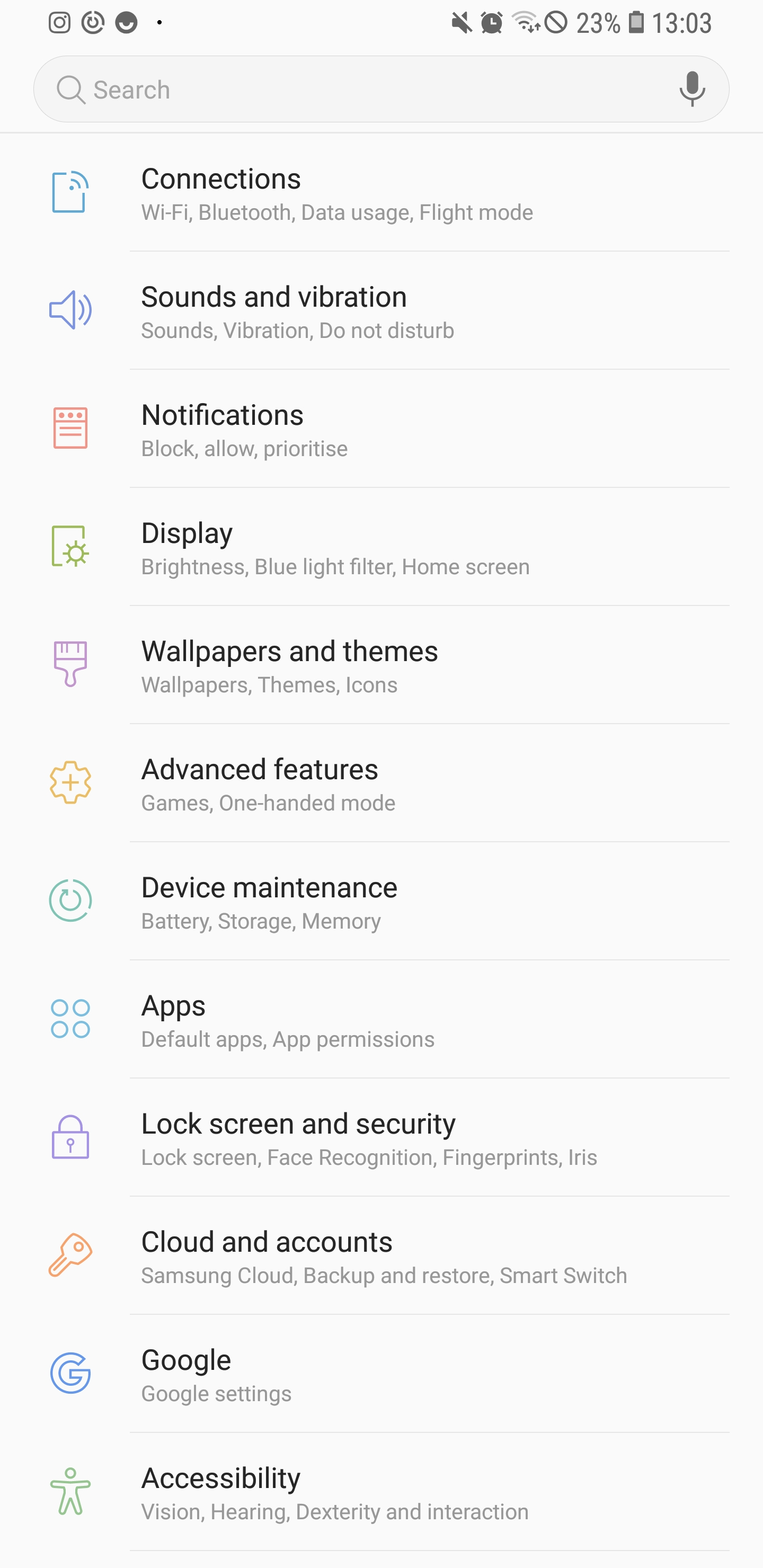This screenshot displays the settings section of a smartphone. The top bar features quick access icons: on the left, shortcuts to the camera and various apps, while on the right are icons indicating the speaker is muted (depicted by a line through the speaker symbol), the current time displayed in military format (13:03), Wi-Fi signal strength, an unknown icon, and a battery level critically low at 23%. 

The main settings menu is shown in a vertical list, encompassing the following categories: Connections, Sounds and Vibration, Notifications, Display, Wallpapers and Themes, Advanced Features, Device Maintenance, Apps, Lock Screen and Security, Cloud and Accounts, Google Settings, and Accessibility. Each category provides access to various customization and configuration options for the device.